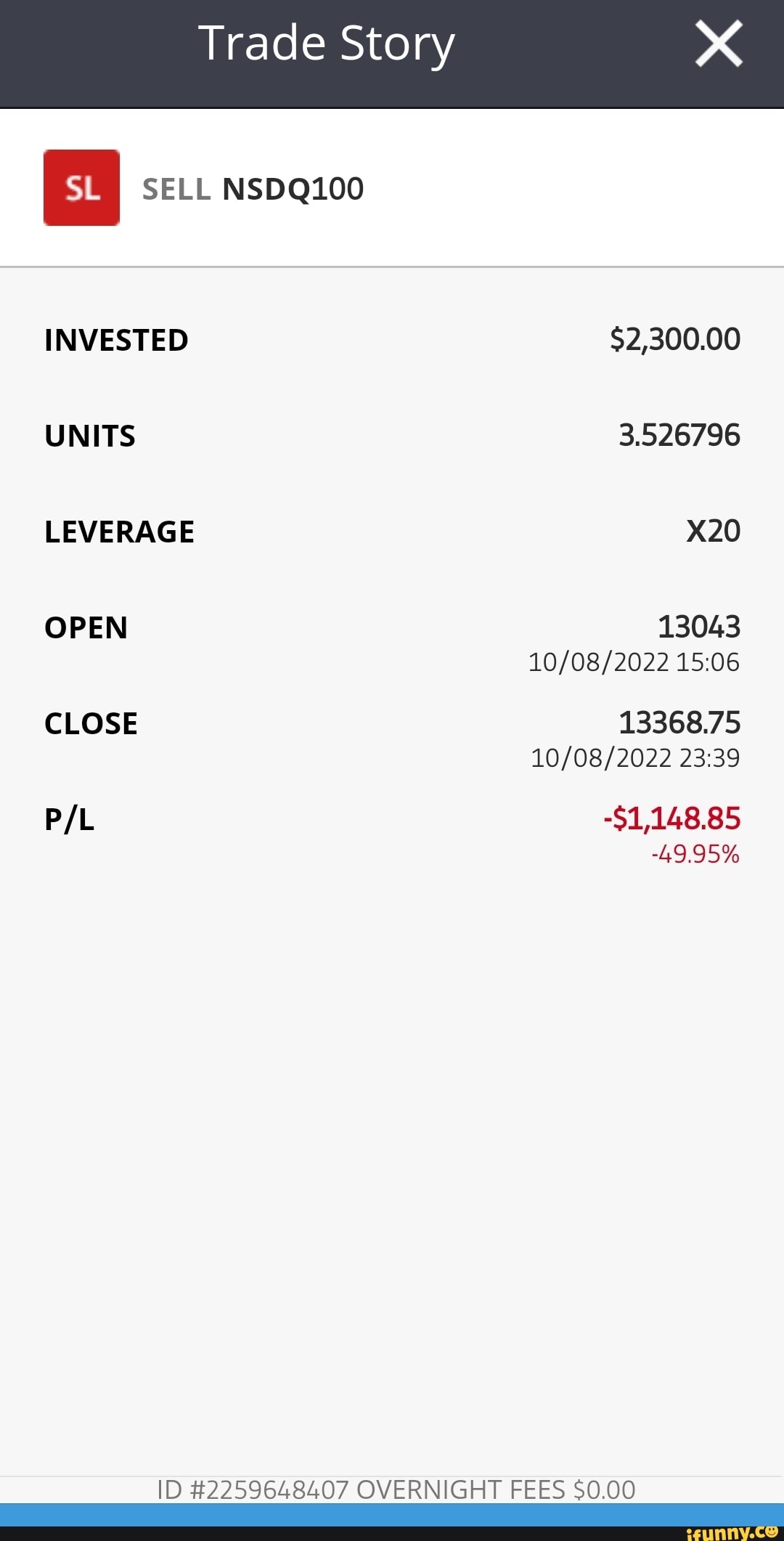This image displays a webpage from an individual's investment account, though the specific platform is not identified. The header, "Trade Story," is prominently displayed in white text on a navy blue background. Below this, the initials "SL" are marked within a red square, indicating a sell order for NSDQ 100.

The account summary shows an investment amount of $2,300, detailing the transaction involved approximately three and a half units, each multiplied by 20. The trade was initiated on October 8th, 2022, at 15:06 and concluded later that day at 23:39.

Financial outcomes are prominently featured: the investor experienced a significant loss of $1,148.85, equating to a negative return of 49.95%. These loss figures are prominently highlighted in red to signify the negative impact.

Surrounding details include a light gray background with most text rendered in black. A blue line demarcates the bottom section of the webpage, where an ID number and a note confirming the absence of overnight fees are also displayed.